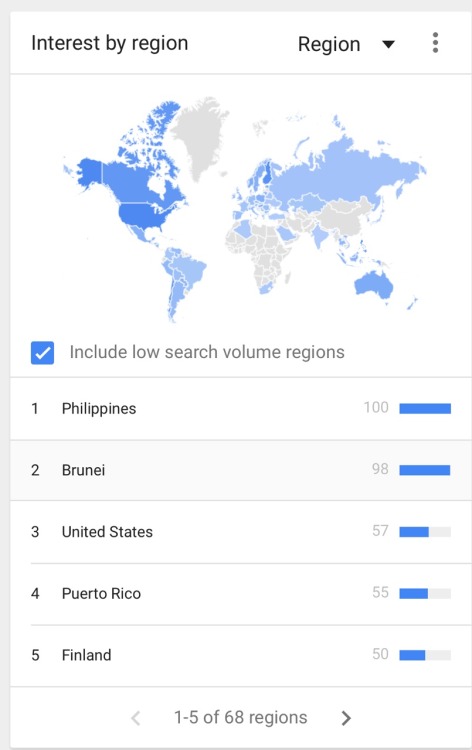The image displays a vertical rectangular box on a white background, featuring a light blue border along the top and left side. At the very top of the image, the title "Interest by Region" is printed in black ink. To the right of the title, there is a dropdown arrow next to the word "Region" and three dots indicating more options.

Below this header, a world map is depicted, highlighting regions in North and South America, Europe, and Africa. These areas are shaded in varying colors: light blue, dark blue, and gray, indicating different levels of interest.

Directly beneath the map, in dark gray ink, is a checked checkbox labeled "Include low search volume regions."

Further down, a vertical list ranks countries by search interest:
1. Philippines (100%) – represented by a full horizontal blue bar.
2. Brunei (98%) – indicated by a nearly full horizontal blue bar.
3. United States (57%) – shown with a horizontal blue bar at 57%.
4. Puerto Rico (55%) – displayed with a horizontal blue bar at 55%.
5. Finland (50%) – marked with a horizontal blue bar at 50%.

At the bottom of the list, text states "1 to 5 of 68 regions," accompanied by forward and back arrows for navigation.